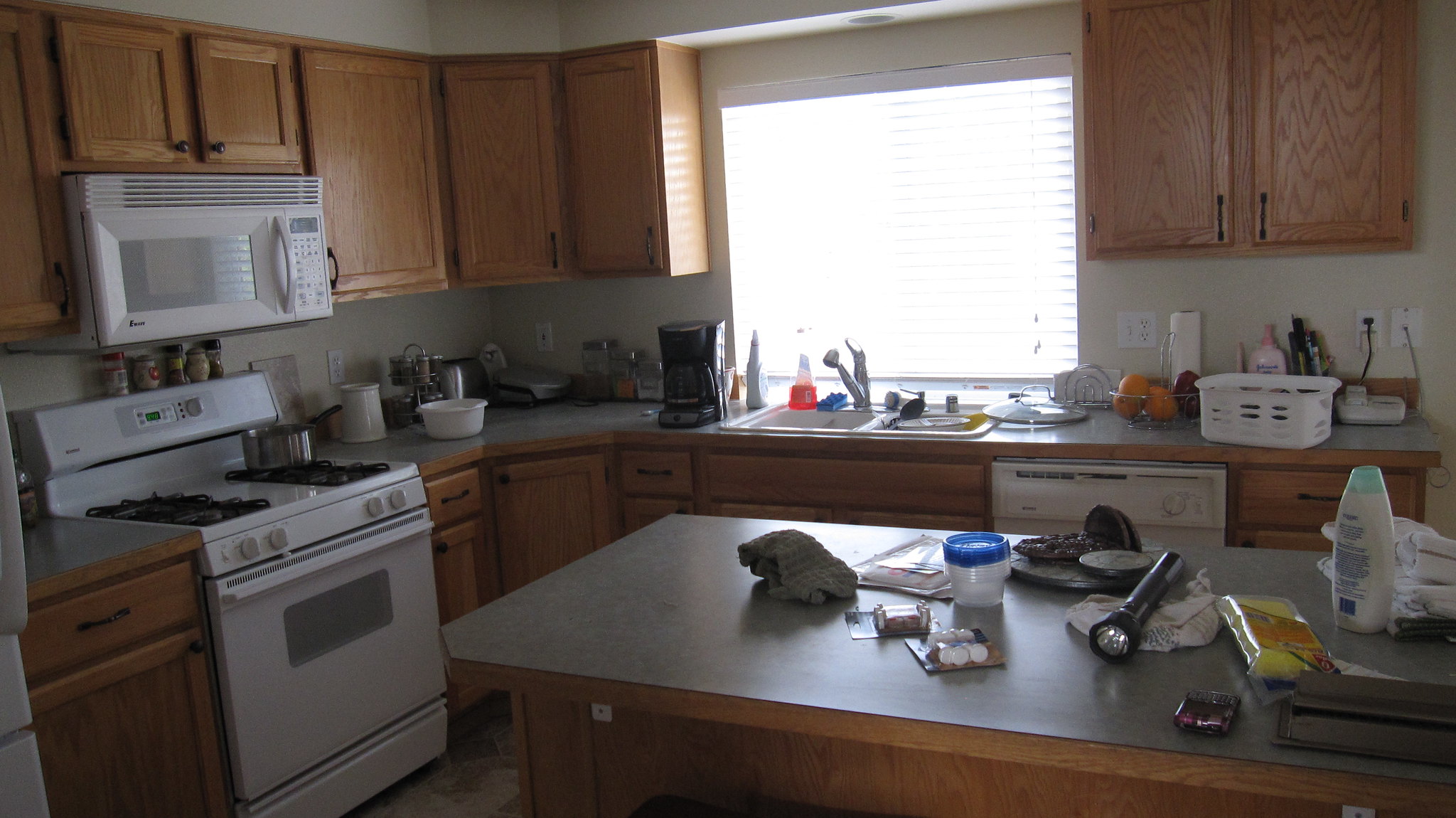This detailed, color photograph captures the interior of a kitchen bathed in daytime light. The kitchen features a central island that matches the wood cabinetry and green countertops. The cabinets are adorned with black handles. On the island, various items such as a flashlight, a bottle of lotion, towels, a cup, and a set of keys are scattered. Behind the island, a row of cabinets is punctuated by a window through which sunlight pours, confirming the daytime setting.

The countertop hosts an assortment of items, including a coffee pot, sink detergent, a lid, a small white basket, and a bowl of fruit containing oranges. To the left of the window, several bowls are arranged, and a stainless steel stove topped with a single pan sits next to them. Above the stove, a microwave completes the kitchen setup.